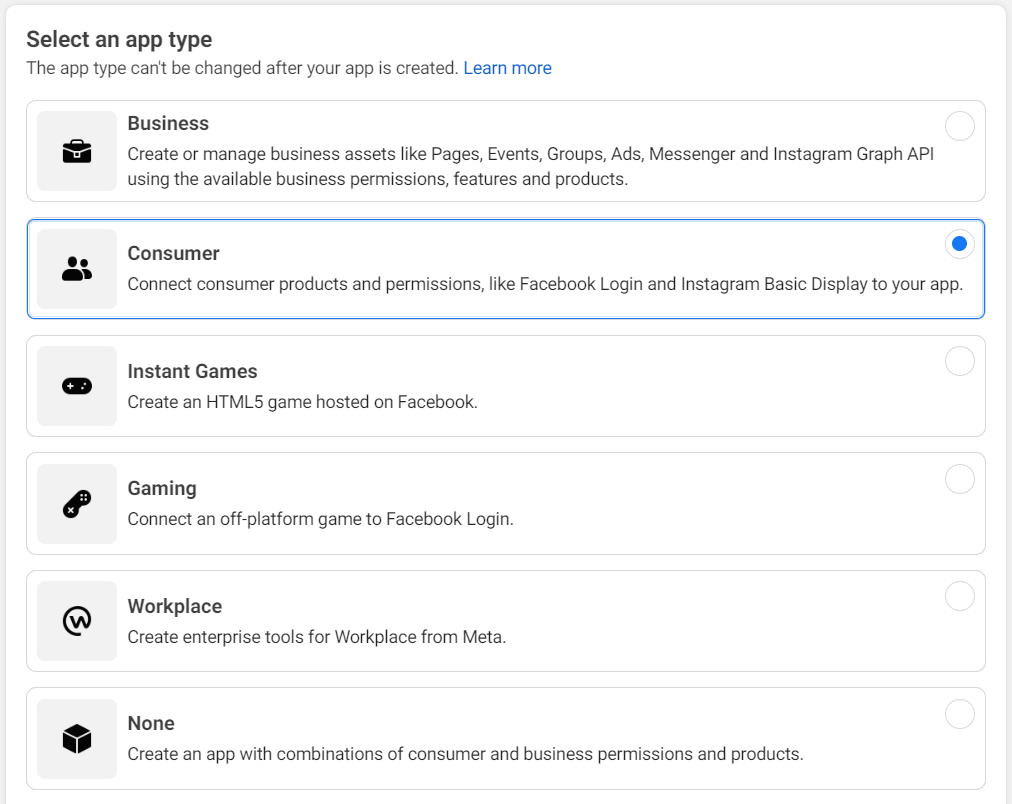The web page features a clean, organized layout with distinct sections and categories to guide the user through the process of selecting an application type. 

At the top left corner, the border is a subtle light gray, transitioning to black. Prominently displayed in this section, the heading reads "Select an App Type" in bold, black lettering. Below this, in smaller gray font, is an important note stating, "The app type can't be changed after your app is created." Adjacent to this note is a clickable link in blue font that says, "Learn more."

Below the introductory section, various app type options are presented. Each option is enclosed within a rectangular light gray border with rounded corners, distinguished by a dot at the top right corner.

1. **Business**: 
   - **Icon**: A briefcase, located to the left.
   - **Description**: In bold black text, "Business" is followed by the detailed explanation in regular font: "Create or manage business assets like Pages, Events, Groups, Ads, Messenger, and Instagram Graph API using the available business permissions, features, and products."

2. **Consumer** (This option is currently selected):
   - **Icon**: Two silhouettes, located to the left.
   - **Description**: "Consumer" in bold black text, followed by the explanation in regular font: "Connect consumer products and permissions like Facebook Login and Instagram Basic Display to your app."
   - **Selection Indicator**: A filled blue circle with a checkmark is visible at the top right corner, with the circle outlined in blue.

3. **Instant Games**:
   - **Icon**: A game controller, located to the left.
   - **Description**: "Instant Games" in bold black text, followed by: "Create an HTML5 game hosted on Facebook."

4. **Gaming**:
   - **Icon**: A slanted game controller, with the plus sign at the bottom left and the ABC controls at the top right, located to the left.
   - **Description**: "Gaming" in bold black text, followed by: "Connect an off-platform game to Facebook Login."

5. **Workplace**:
   - **Description**: "Workplace" in bold black text, followed by: "Create enterprise tools for Workplace by Meta."

6. **None**:
   - **Description**: "None" in bold black text, followed by: "Create an app with combinations of consumer and business permissions and products."

This detailed and structured layout ensures users can easily navigate through the options and make an informed decision about the type of application they wish to create.